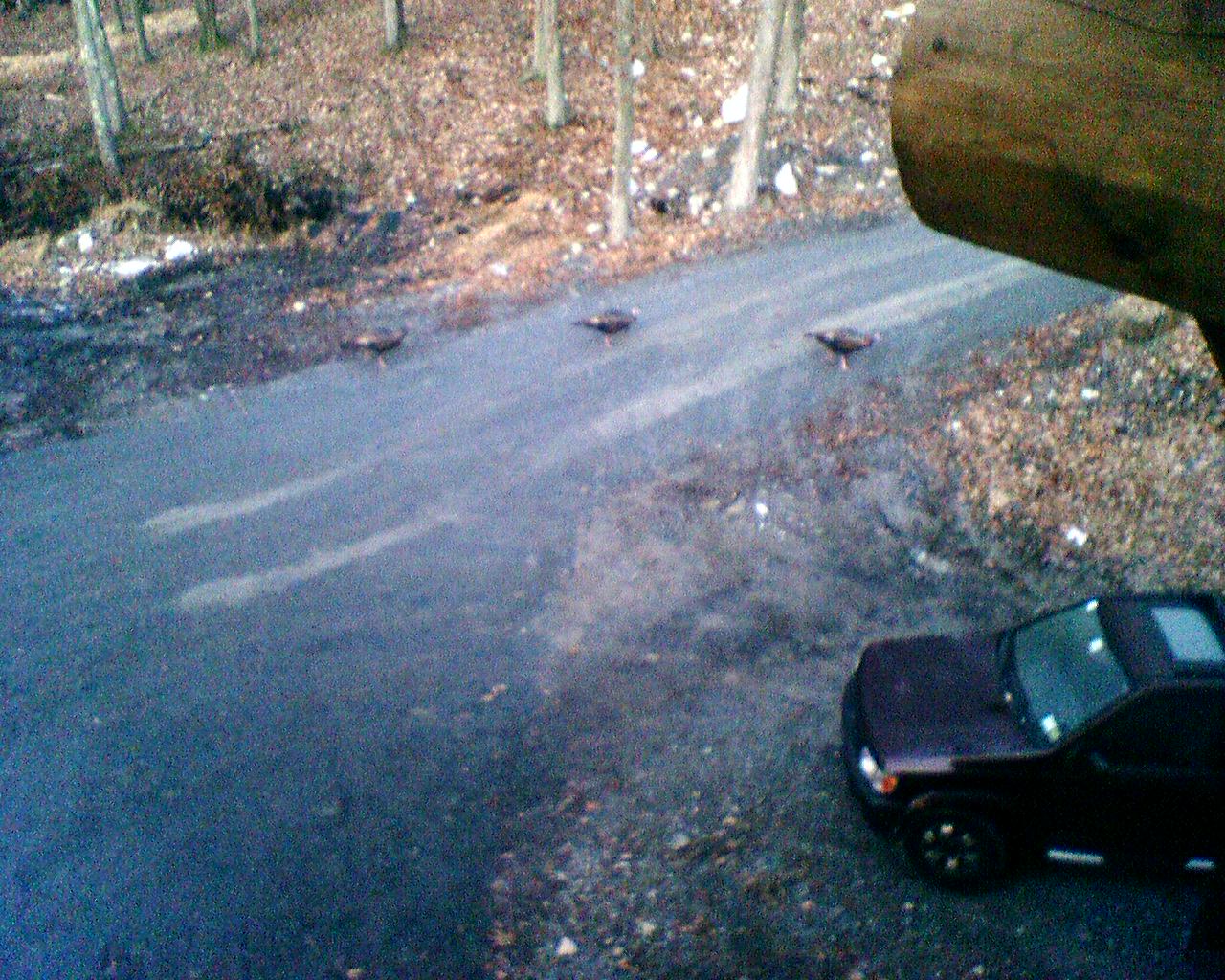The aerial image, resembling a view from a security camera, captures an outdoor scene during a rainy day. Dominating the lower right corner is a driveway that merges into a gravel road, where a wet, purple vehicle with a sunroof is parked, facing left. Above the driveway, extending into the upper right corner, is a piece of lumber, likely part of a house roof. In the distance, the bottom parts of skinny trees are visible, standing among thousands of scattered brown leaves. Three turkeys, distinguished by their dark brown bodies and slender pink legs, are crossing the road in a line. One turkey is nearing the vehicle, another is in the middle of the road, and the third is almost at the far side, marking their path across the gravel amidst the rainy, leaf-strewn landscape.